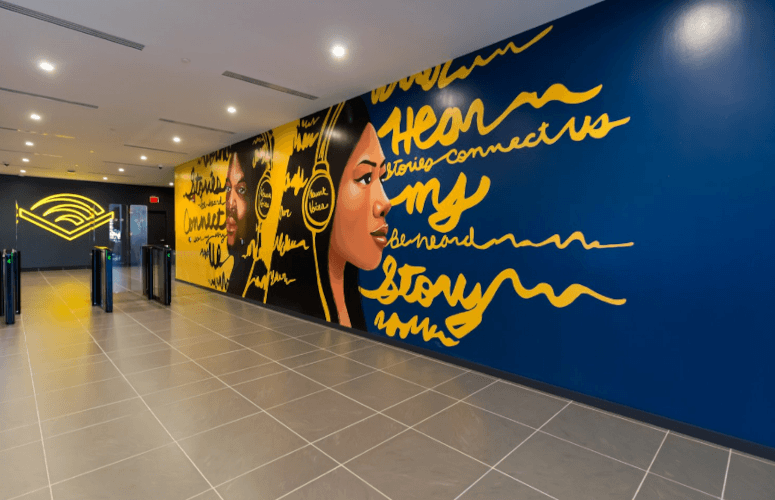The mural inside the building appears to serve as an inviting focal point, likely situated near the entrance of a theater or auditorium. The expansive artwork spans a wall that climbs to a height of approximately 10 to 15 feet and stretches horizontally to a length at least five times its height. Dominated by vibrant hues of yellow, blue, and black, the mural features two prominent figures. On the left, there's a man who resembles Will Smith, donning headphones, while on the right, a woman, also wearing headphones, emerges from the blue background. Both figures are rendered with a sense of vitality against the mural's contrasting yellow and blue backdrop. The mural is adorned with cursive text, highlighted in yellow, which includes phrases like "Here stories connect us" and "Be heard," emphasizing themes of unity and storytelling. Adjacent to this striking visual are functional elements of the building's entrance—automated security gates, indicating entry with green lights, and polished wooden floors with white patterns. Above, the ceiling features geometric gray patterns with embedded LED lights, contributing to the modern ambiance of the space. Further in the background, a glass door adorned with a red entry or exit symbol hints at the building's dynamic flow of visitors.